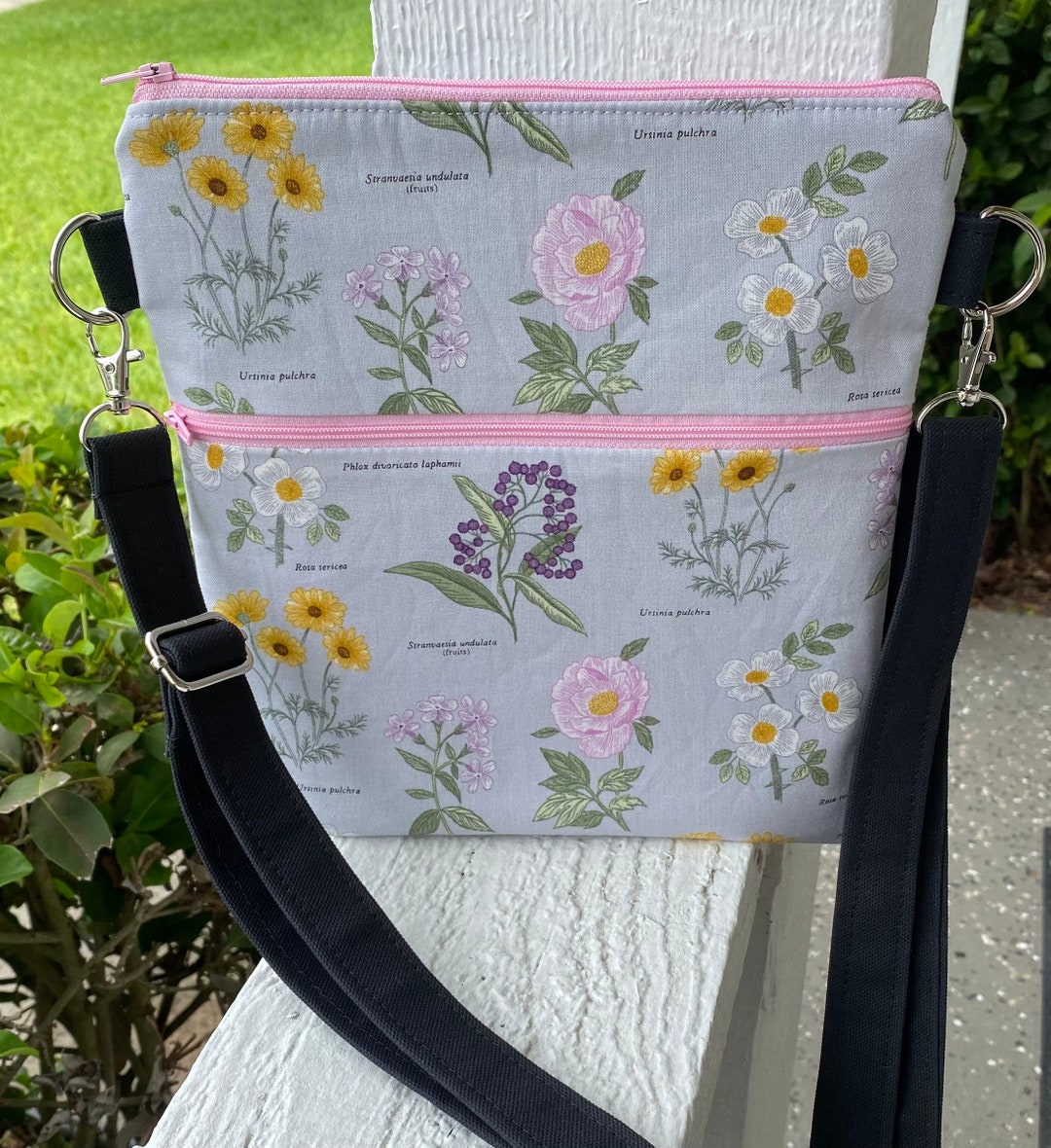The image shows a floral-patterned shoulder bag placed on a ledge, which appears to be part of a porch or a white-painted wooden fence. The bag is adorned with various colored flowers and features two pink zippers: one across the top and another about a quarter way down. Its black adjustable strap, attached with spring-loaded hooks, extends down to the bottom right corner of the image. The background includes a leafy bush and a green grassy area to the left, while the right side of the image shows a cement surface. The overall setting is outdoors, providing a glimpse of a serene porch environment.